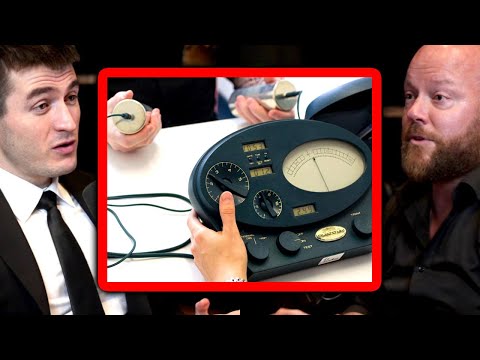This composite image consists of three photos set against a black background, depicting a scene from a podcast, likely the Lex Friedman show. On the left, Lex Friedman, easily identifiable by his spiky brown hair, is dressed in a classic black suit, white collared shirt, and black tie. Opposite him on the right side is Alex Jones, characterized by his bald head, reddish beard, and an open-collared black shirt. Positioned between their photos is an image showing a lie detector-like device, which is central to the scene. The device appears to be a black oval at the top evolving into a box with numerous dials, digital screens, and needles, all connected by wires. The hands of one individual are seen grasping the cylindrical metal-topped sensors connected to the device, while another set of hands manipulates the machine, indicating the monitoring of readings possibly related to a polygraph test or similar device.